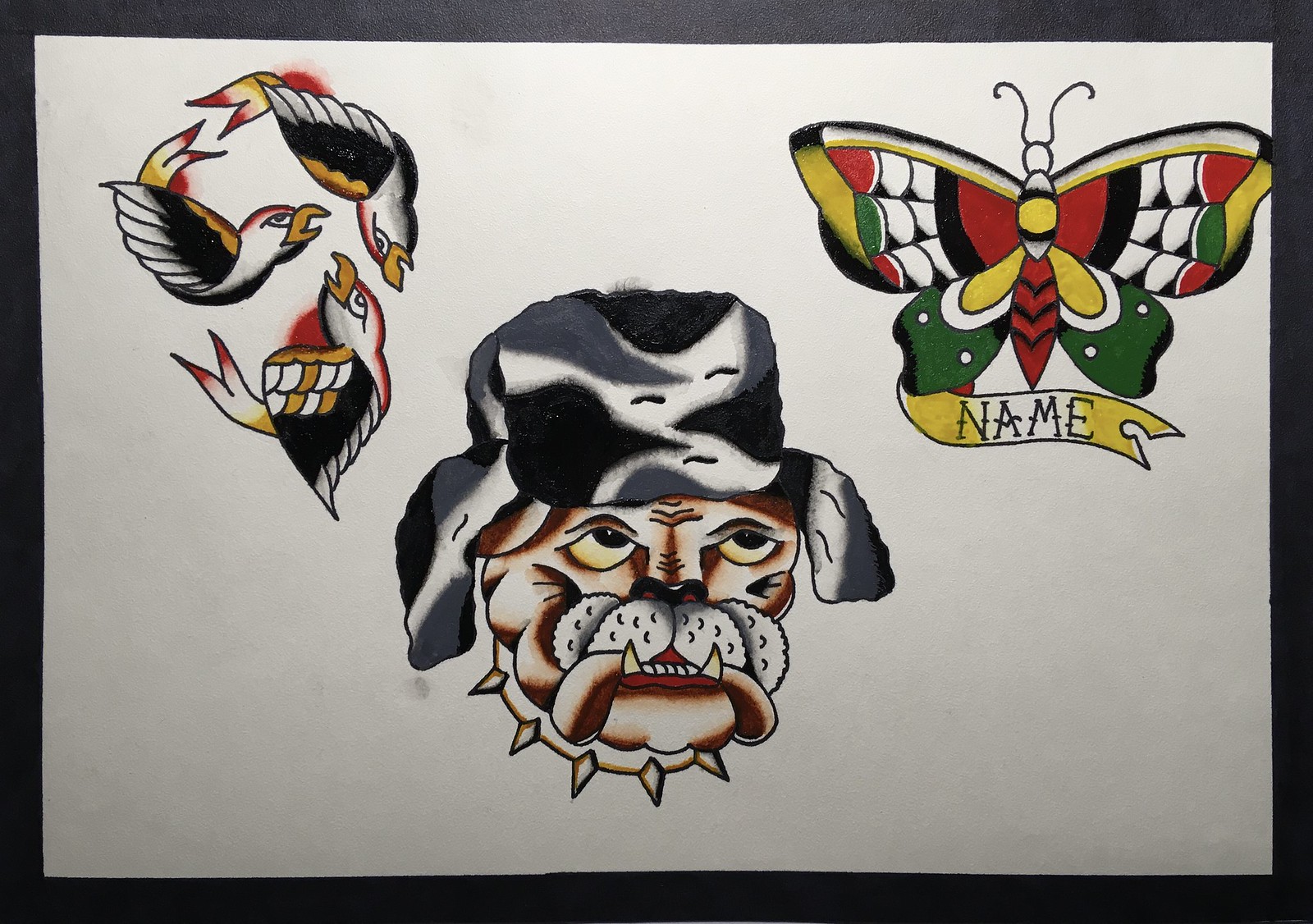The image depicts a white sheet of paper in a landscape orientation, placed on a black mat, showcasing three distinct tattoo flash designs. In the upper left corner, there's an intricate illustration of three birds with yellow beaks, yellow and white wings, and longer tails that end in two points. The birds are arranged in a semi-circular manner, creating the illusion of a face at first glance. In the upper right corner, there's a vibrant butterfly that features red, black, dark green, and yellow hues. The butterfly holds a trailing yellow banner below its wings with the word "NAME" inscribed in black letters. Dominating the lower center of the sheet is a detailed depiction of a bulldog. The bulldog is characterized by its brown and tan fur, prominent eyes, a sharp-toothed studded collar, and a green and black hat with ear flaps. The entire sheet exudes an old-school tattoo flash style, unified by a black border.